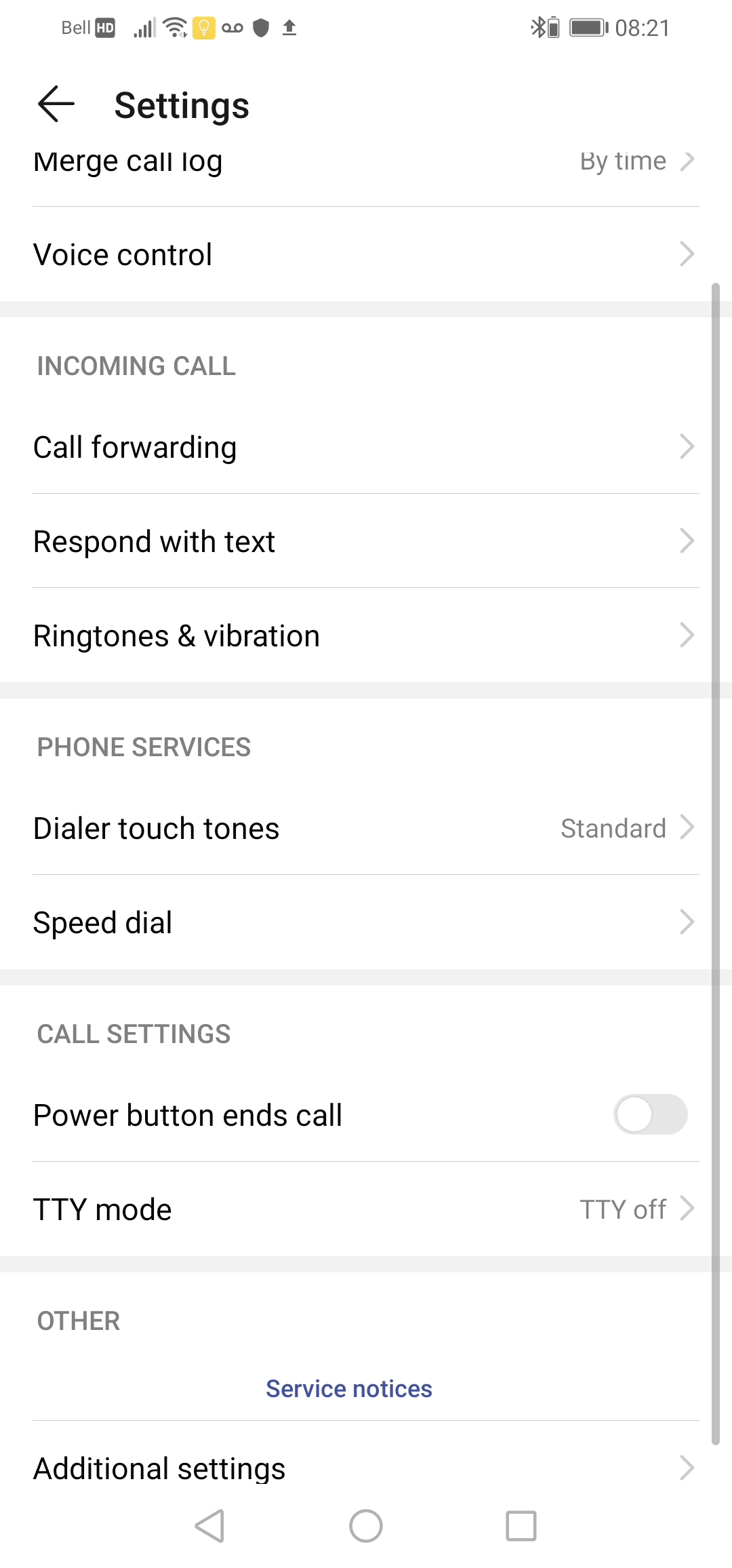Screenshot of a Settings Page on a Phone

The screenshot captures a portion of the settings page on a cell phone, displaying various configuration options against a white background. At the top, the word "Settings" is prominently displayed in black letters, accompanied by a left-pointing arrow, suggesting a navigation option to go back.

The page has been scrolled down, partly cutting off the words "Merge call log by time" and "My time" at the top, with portions of the letters no longer fully visible.

Below are several sections organized by thick gray dividers:

1. **Voice Control**
   - A left-pointing arrow next to "Voice Control" follows this section label, indicating further navigation options.

2. **Incoming Call**
   - This section is marked in bold gray letters. Under it, various call settings are listed:
     - Call Forwarding (with a left-pointing arrow)
     - Respond with Text (with a left-pointing arrow)
     - Ringtones (with a left-pointing arrow)
     - Vibration (with a left-pointing arrow)

3. **Phone Services**
   - The next section, also separated by a thick gray bar, includes:
     - Dialer Touch Tones: Set to "Standard" with a gray arrow beside the setting.
     - Speed Dial: Indicated by a gray arrow.

4. **Call Settings**
   - Under this category:
     - Power Button Ends Call: Featuring a toggle button currently switched off.
     - TTY Modes: Displaying "TTY Off".

5. **Other**
   - The final section, simply labeled as "Other," contains the centered text "Service Notices."

The arrangement and partitioning make it clear where different settings are grouped, aiding in navigation and adjustment of the phone's features.